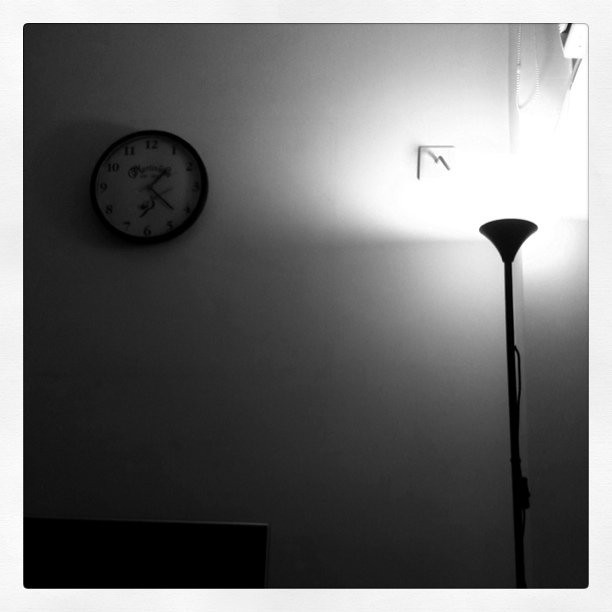The image depicts the interior of a dimly lit room rendered in black and white. On the left side of the white, scuffed wall hangs a round clock with a black circular frame, white face, and black numerals and hands. The clock casts a shadow to the left, and although the design on its face is partially obscured by the darkness, the time reads 1:23. Below the clock, barely visible due to the low lighting, is a piece of furniture. On the right side stands a tall, black floor lamp with a pole base that flares out at the top, resembling a funnel. The lamp's halogen light shines upwards, casting a warm glow on the ceiling and illuminating part of the room. To the right of the clock and partially illuminated by the lamp, there is a metal object, possibly a hat rack or hook. Above the lamp, there might be a balcony, suggested by shadows and shapes barely discernible in the dim environment.